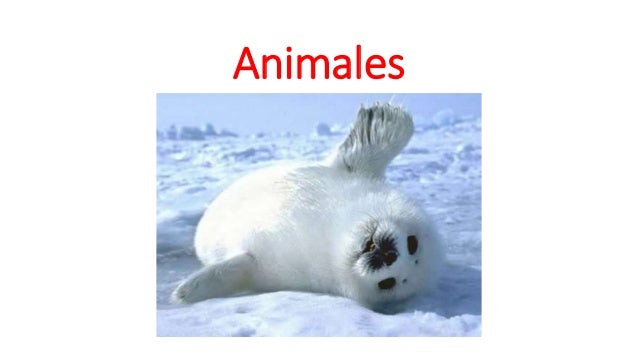In this detailed photograph, a white, fluffy harp seal is lying on its back in the snow, with one flipper raised and the other resting on the ground. Its body is covered in fuzzy fur, and its pure black eyes stare directly forward. The seal’s head is tilted halfway upside down, displaying a black nose set amidst a facial area that contrasts with its white fur. Its black mouth is slightly open, revealing a white outline around the edges. The entire scene is set against a snow-covered landscape with varying levels of snow. In the distance, the horizon line is visible about one-eighth down from the top of the image, with a clear blue sky above. Above the photograph, there is red text spelling out "A-N-I-M-A-L-E-S," with the first letter capitalized and the rest in lowercase.